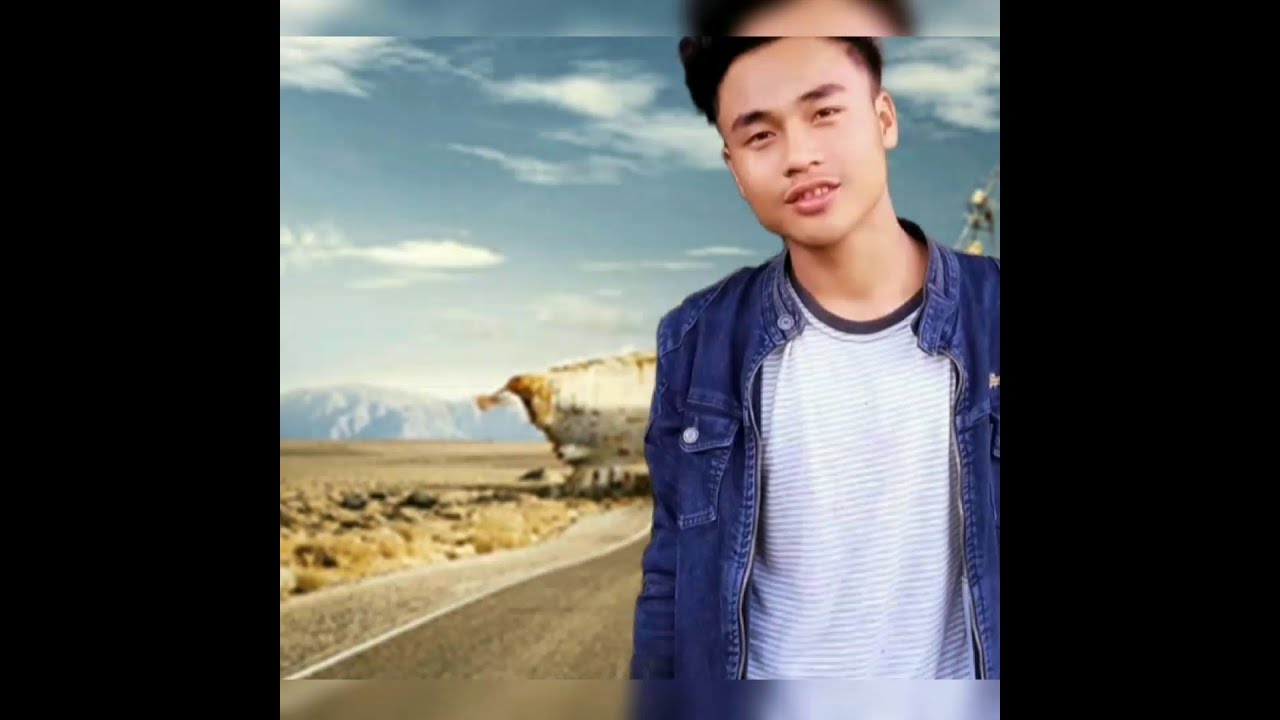The image features an Asian male, wearing a dark blue denim jean jacket, unzipped to reveal a thin-striped white and light gray shirt with a black collar. He has short black hair, shaved thin on the sides and taller on top, and black eyebrows. He stands offset to the right side of the photo, subtly smiling. The background depicts a blue sky filled with thin, white clouds, and a distant gray mountain range. The setting appears to be a desert environment with a partially visible paved road, sand, and some tan-colored bushes. There's also a mysterious large object with legs, resembling a landed ship, and some people near it. The photo has black rectangular frames on the sides and additional framing lines above and below, suggesting that the image might have been digitally altered or superimposed onto the background.